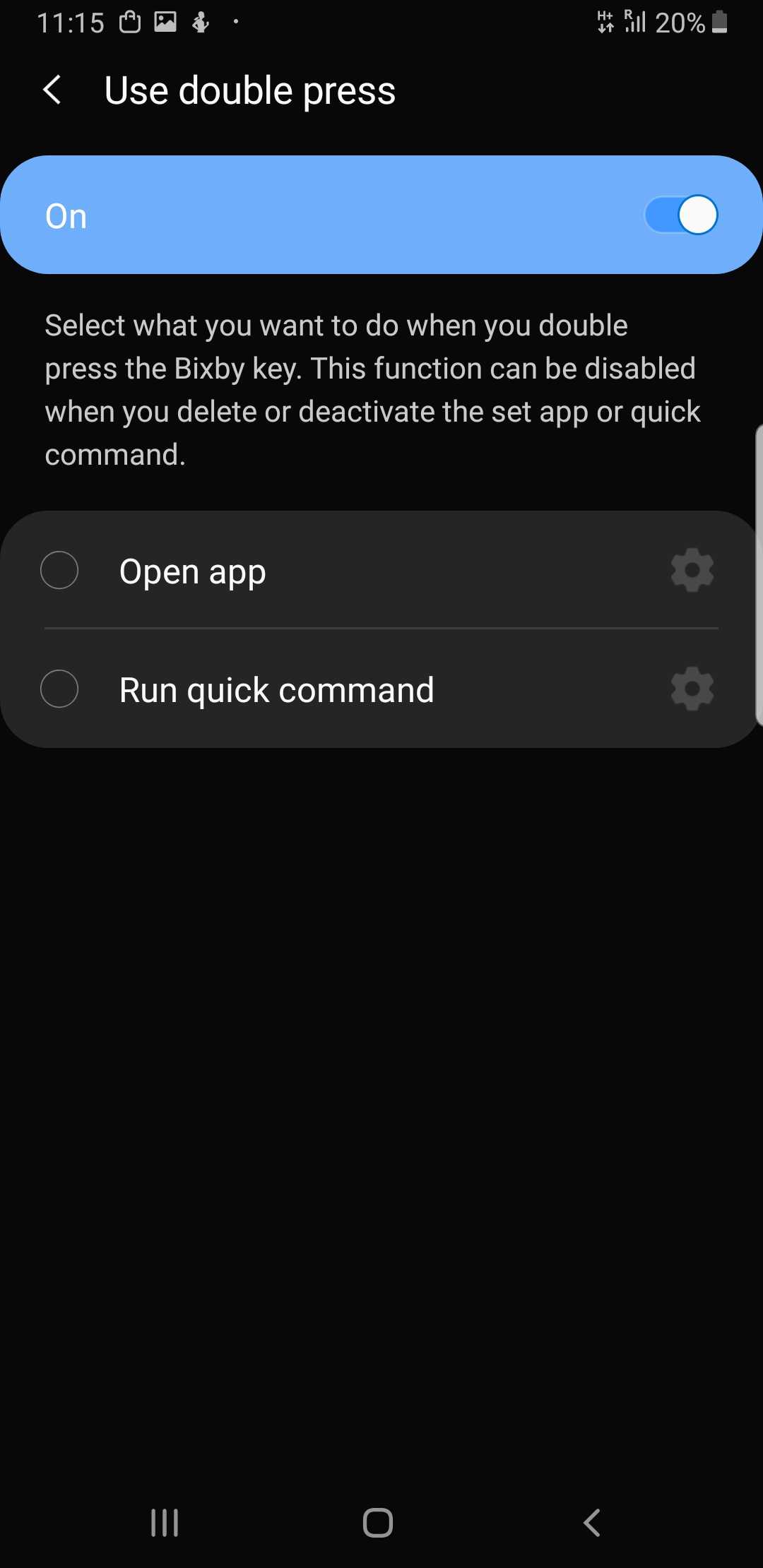This image depicts a screenshot from a smartphone, featuring a black background. The top left corner displays the time as 11:15, alongside 4 signal bars and a battery icon showing 20% remaining. Beneath this, a back arrow symbol is present. The main content shows a blue box with the word "On" on the left and a toggle switch on the right, which is currently activated.

Below the blue box, gray text reads, "Select what you want to do when you double press the Bixby key. This function can be disabled when you delete or deactivate the set app or quick command." Under this instructional text is a gray box with two radio buttons.

The first radio button, labeled "Open app," is accompanied by a settings gear icon on the right. The second radio button is labeled "Run quick command" and also includes a settings gear icon on its right-hand side. The lower part of the screen is mostly empty, with navigation symbols at the bottom, including three vertical lines, a square, and a less than symbol.